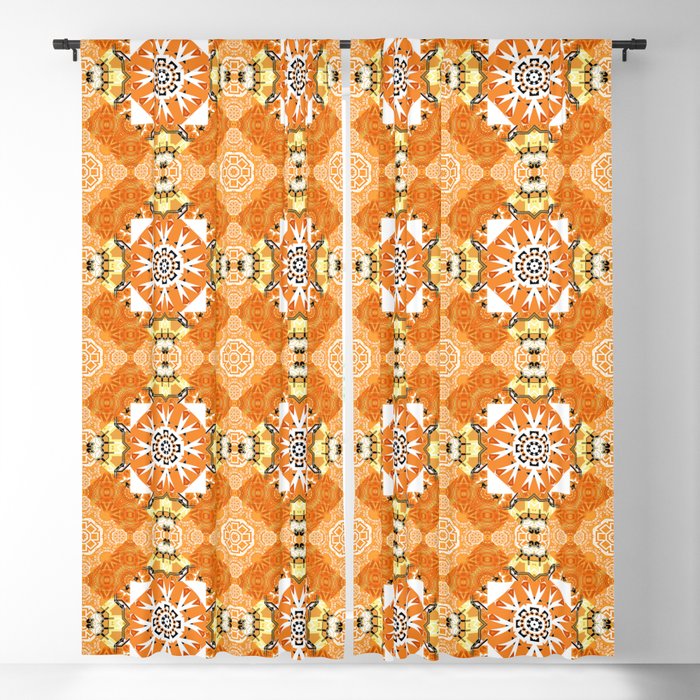The picture displays an elaborate curtain set hung on a black curtain rod, featuring two panels with a Southwestern and Native American-inspired design. Dominated by striking geometric patterns, the fabric showcases a vivid array of colors, including bright orange and yellow with accents of white, blue, brown, and hints of black and red. Each panel hangs straight down and is made from a heavy material, creating a bold and vibrant aesthetic. The design includes elements reminiscent of Mayan symbols, including white squares with sun-like motifs. These eye-catching curtains, with their intricate and repetitive patterns, stand out against a white wall, making for a visually dynamic display.